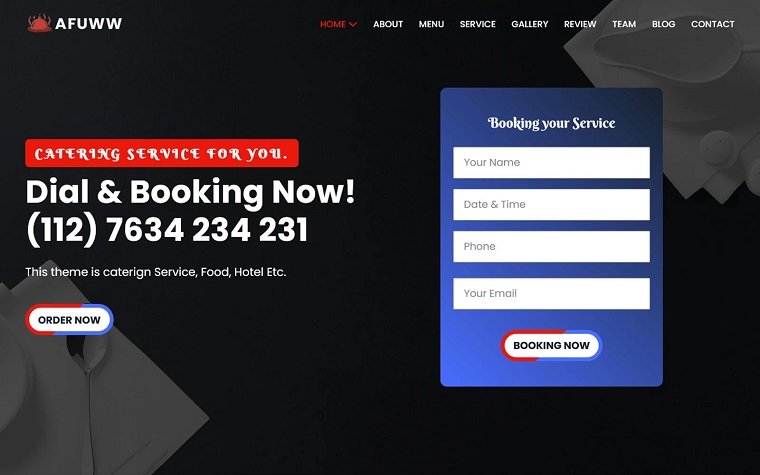The image is a screenshot of a webpage with a predominantly dark gray, almost black background. In the bottom left-hand corner, there is a slightly visible white napkin with a silver spoon atop it, possibly alongside a cup. The top right-hand corner of the image contains another folded napkin and what appears to be a cream holder or a cream server bowl. Scattered across the image are small white dots.

In the top left-hand corner, "AFUWW" is written in white text next to a red icon of a covered dish with steam rising from it. The top right-hand corner of the webpage contains a navigation menu with the following options: Home, About, Menu, Service, Gallery, Review, Team, Blog, and Contact.

On the left-hand side, there is a red button labeled "Catering Service for You," and below it, the text "Dial and Booking Now" followed by the phone number "112-7634-234-231." 

Additionally, the theme of the website is indicated as Catering, Service, Food, Hotel, etc. There is an "Order Now" option available. 

On the right-hand side, a blue rectangle houses a "Booking Your Service" section with input forms for your name, date and time, phone number, email, and a "Booking Now" button.